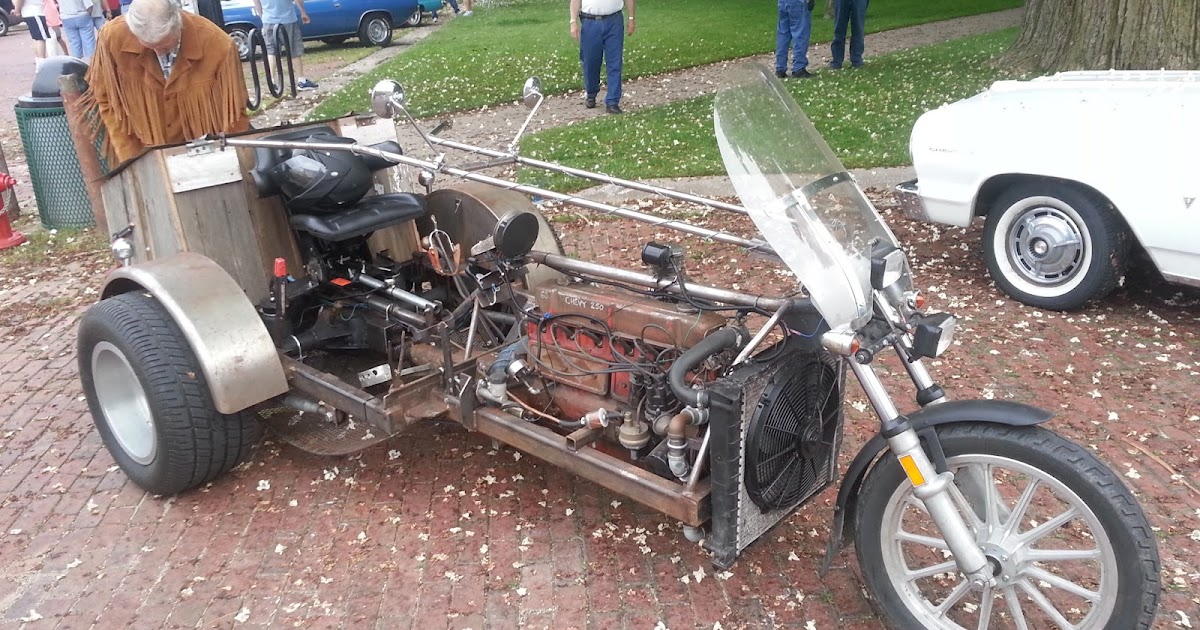The image features a unique, custom-built vehicle resembling an old-fashioned motorcycle with a three-wheel design. The front end displays a classic motorcycle appearance, including a single headlight centered within a wheel guard and a windshield. Directly behind the front wheel, there is an exposed engine equipped with a cooling fan. The seat, situated further back aligned with the two thicker rear wheels, contributes to a considerably elongated structure compared to a standard motorcycle. Behind the seat, there is a large rectangular storage box, and a man, identifiable by his gray hair and brown suede jacket with tassels, is interacting with this box. The scene appears to be part of a gathering or car show, as suggested by the scattered people in blue jeans—one in shorts—partially visible in the background. Additionally, a white classic car and a thick tree are positioned to the right of the vehicle, with another classic blue car discernible at the upper left. The pavement beneath the vehicle is constructed of reddish-brown bricks, covered with numerous small flower petals likely from the nearby tree. A green garbage can is also visible to the left. Grass and a sidewalk extend into the background beyond the tree and classic cars.